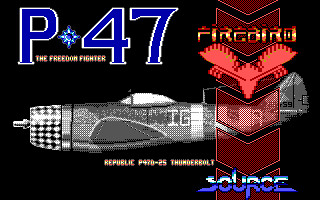A sleek silver fighter jet, reminiscent of a video game graphic, is displayed against a stark black background. The jet, viewed from the side, showcases a shiny domed cockpit and a streamlined, futuristic design. At the top left corner of the screen, the text "P-47" is prominently featured in bright blue letters and numbers with a white border. Next to it, in striking orange and yellow letters, the word "Firebird" is displayed. Several translucent red arrows point downward, overlaying the scene. In the bottom right corner, the word "Source" appears in blue and white. Below the jet, in small white letters, the inscription "Republic P-970-25 Thunderbolt" is visible, providing further detail about the aircraft.